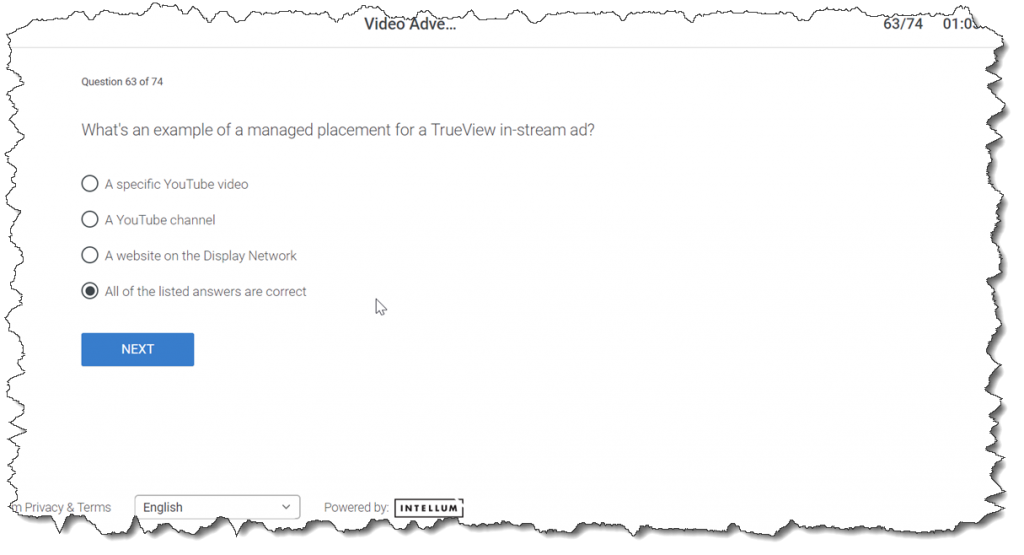A screenshot appears to be digitally altered to resemble a piece of paper with jagged, hand-cut edges, giving it a unique, sketch-like appearance. In the top-right corner, partially cut-off text reads "63/74 01:20" alongside the phrase "video ad v...". A long, gray horizontal line stretches across the image, serving as a visual divider. Below this line, the text "Question 63 of 74: What's an example of a managed placement for a TrueView in-stream ad?" is prominently displayed. Four multiple-choice options are listed, each accompanied by a circular checkbox. The options are:
1. A specific YouTube video
2. A YouTube channel
3. A website on the Display Network
4. All of the listed answers are correct

The fourth option is selected, indicated by a filled black circle. Beneath the options, a blue "Next" button with white text appears, inviting the user to proceed. In the bottom left corner, partially visible text shows an "M," followed by "privacy and terms." There’s also a language selection box labeled "English" with a clickable arrow for changing settings. The image is marked "powered by Intellim" at the bottom, denoting its origin.